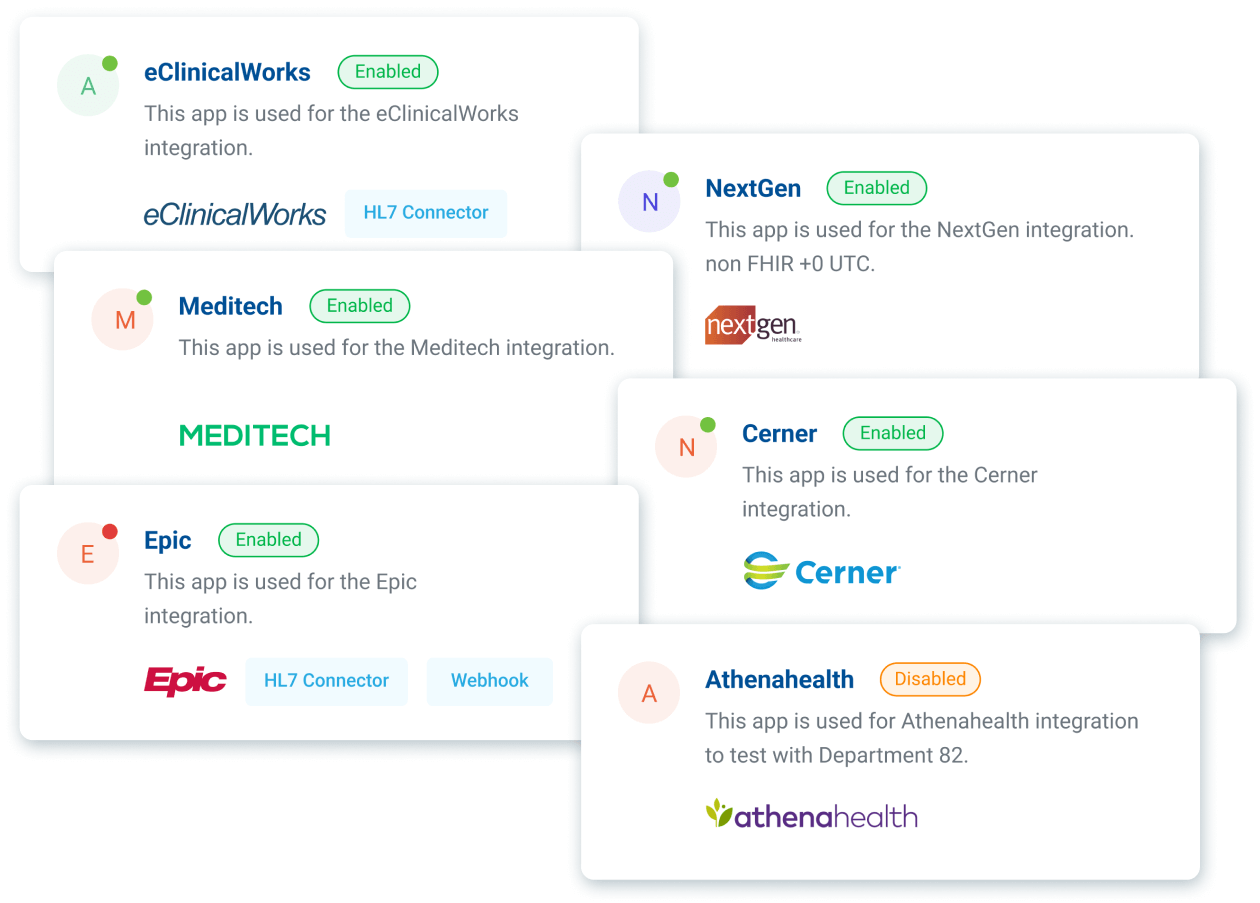Screenshot Description: Integration Apps Interface

The screenshot appears to be part of a website, showcasing various integration applications through a series of overlapping rectangular cards, positioned diagonally. The background is white, and the cards are grouped into two columns: three on the left and three on the right. Each card features a circular icon with a green dot in the upper left corner, signifying an enabled status.

Left Column:
1. **eClinical Works Integration (Enabled)**
   - **Card Color:** Green
   - **Description:** This app is used for eClinical Works integration, featuring the eClinical Works and HCL connector logo.
   - **Status:** Enabled

2. **Medtech Integration (Enabled)**
   - **Card Color:** Not specified
   - **Description:** This app is used for Medtech integration, identified by the Medtech logo.
   - **Status:** Enabled

3. **Epic Integration (Enabled)**
   - **Card Color:** Not specified
   - **Description:** This app is used for Epic integration. At the bottom, it mentions the Epic HL7 connector and webbook.
   - **Status:** Enabled

Right Column:
1. **NextGen Integration (Enabled)**
   - **Card Color:** Not specified
   - **Description:** This app is used for NextGen integration, described as "non-FHR plus zero UTC."
   - **Status:** Enabled

2. **CIMR Integration (Enabled)**
   - **Card Color:** Not specified
   - **Description:** This app is used for CIMR integration, with the CIMR logo displayed at the bottom.
   - **Status:** Enabled

3. **Athena Health Integration (Disabled)**
   - **Card Color:** Not specified
   - **Description:** This app is used for Athena Health integration, specifically for testing with Department 82.
   - **Status:** Disabled

Overall, the interface seems to be targeted at backend users, possibly administrators or developers, managing various healthcare-related application integrations. The presence of technical terms and specific logos indicates this is not a consumer-facing tool, but rather a specialized utility for integrating and managing different healthcare software systems.